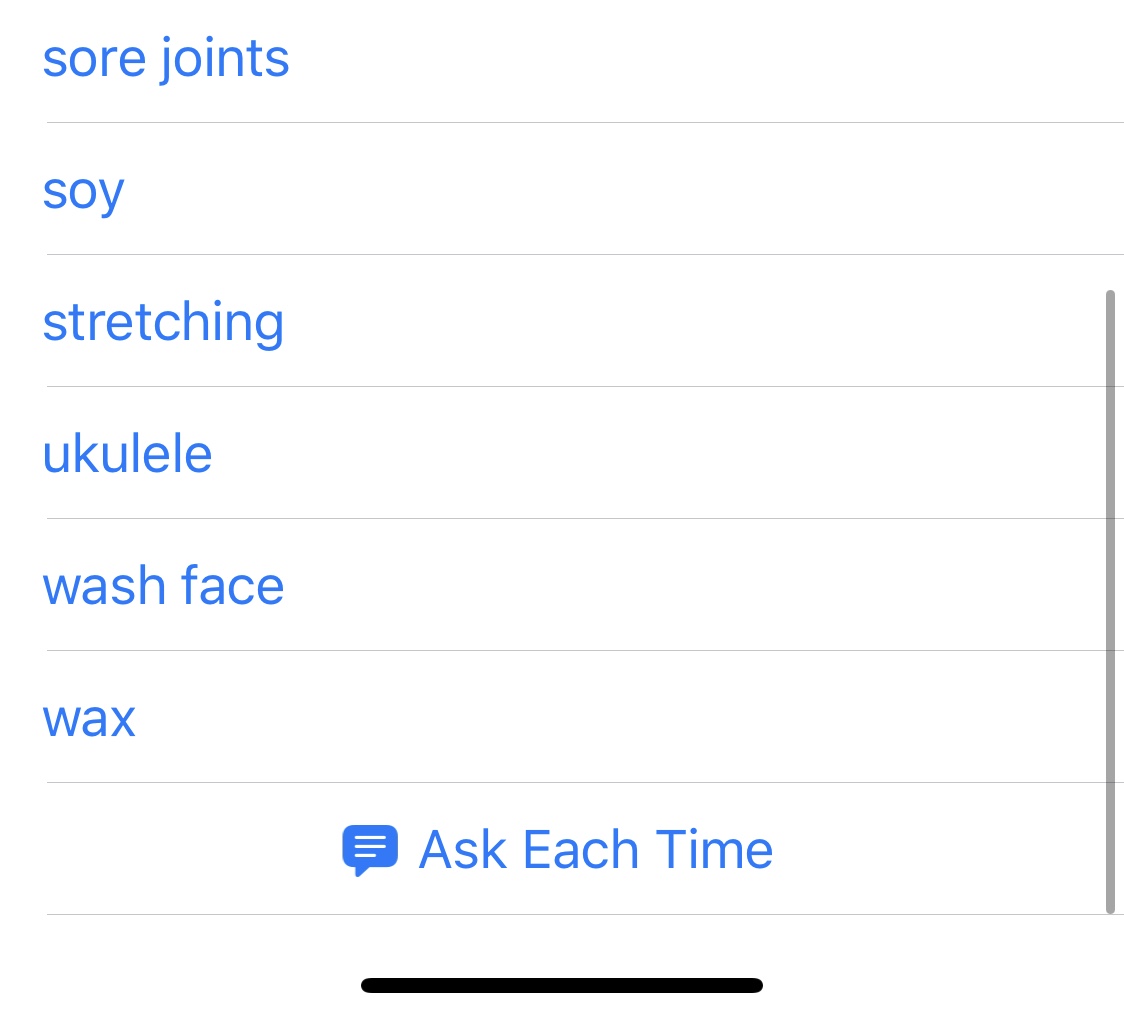This image is an enlarged portion of a web page, showcasing a series of text entries separated by gray lines. The text appears in blue and is listed in a vertical order as follows: "Sore joints," "Soy," "Stretching," "Ukulele," "Face wash," and "Wax." Below these entries, there is a distinct blue conversation box icon labeled "Ask each time," featuring white lines. On the right side of the image, a gray scroll bar indicates that the page can be navigated further. Additionally, a black home bar is located at the bottom of the image. The overall composition suggests that this section has been cropped from a larger web page interface.